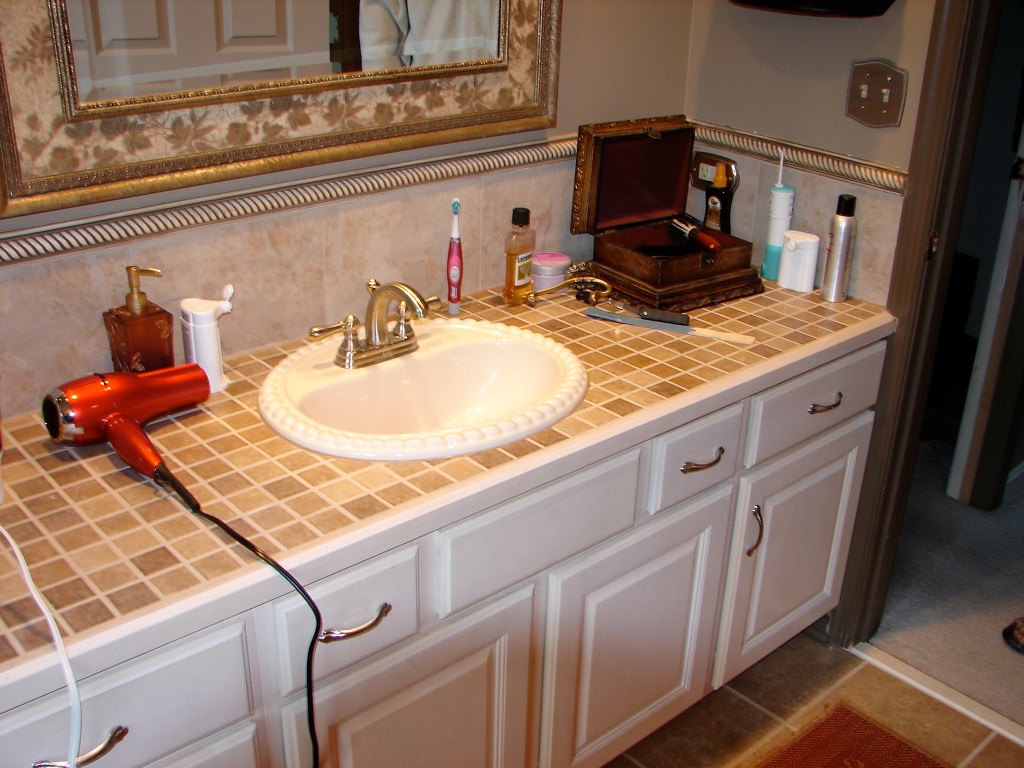This image captures a detailed view of a bathroom, showcasing an intricate mix of design elements and items. A brown door leads into the bathroom, which features gray walls and gray tiles. At the entrance, a brown shoe with a black sole is partially visible. The floor is adorned with large brown tiles and a matching brown mat.

The vanity area is composed of white cabinets with silver handles, arranged with four drawers across the top and four cabinets below. On the wall, a dual light switch with a silver plate is installed. A small shelf hangs on a light brownish-pink wall accented with golden trim. The backsplash features a blend of brown and white tiles, complementing the multi-shaded brown-tiled countertop.

A white, rounded sink with silver faucets is centrally positioned. Adjacent to the sink, there's a red blow dryer with a black cord alongside a white cord. The sink area is cluttered with various items, including a brown pump bottle with a golden pump top, a smaller white pump bottle possibly containing soap, and an electric toothbrush with pink and white coloring. Additionally, a brown bottle of mouthwash with a black cap, a pink makeup item, a long rod, some small gold jewelry, and an open wooden box filled with bottles are scattered across the countertop. A large mirror with a brown leafy print frames the background.

The overall scene portrays a blend of earthy tones and functional items, capturing both the aesthetic and practical aspects of the bathroom.